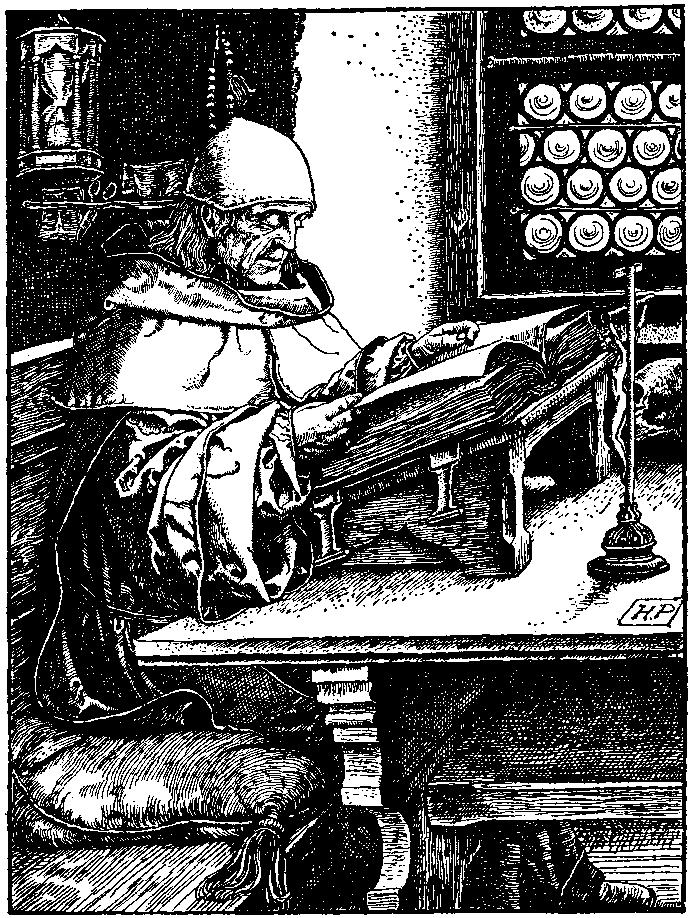The image showcases an intricate, black and white pen and ink drawing evocative of an old, meticulous painting or etching. At its center, a monk or holy figure is depicted seated on a cushioned wooden bench. Clad in a voluminous, layered robe with a white collar, the monk dons a distinctive flat, white cap. He is absorbed in reading an imposing tome set upon a stand on an ornate table. The book, marked with two buckles, suggests it is often locked or securely closed. To the right and on the table, the initials "HP" are prominently visible, possibly indicating the artist's signature. Above the monk, in the upper part of the image, a window or shelf holds several circular objects, which could be old manuscripts or scrolls. Additional elements include an hourglass in the top left corner and what looks like an incense holder or candle, aiding the monk's reading. The background features a stark black wall, adding contrast and depth to the scene.